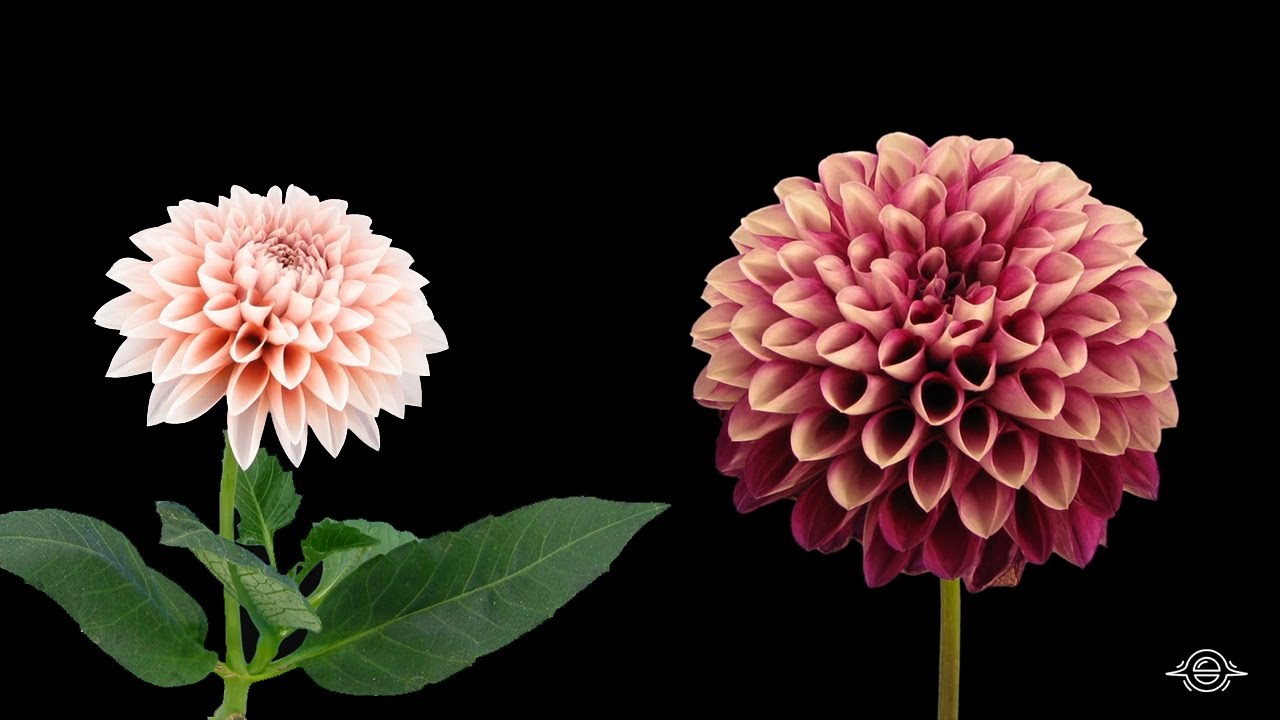In this photograph set against a black background, two flowers are prominently featured, presented within a rectangular frame that is taller than it is wide. The flower on the left is smaller, with light pink petals that are delicately organized in neat circular layers, resembling little cups. It has several green leaves sprouting from its stem. In contrast, the flower on the right is larger and displays rich, dark pink petals, possibly with hues of magenta, arranged in similarly orderly layers, though no leaves are visible around its stem. This flower seems to be pointing diagonally up and towards the right. In the lower right corner of the image is a circular logo with a horizontal line through it, resembling the symbol of a hamburger, accentuated with white curves against a black background. This photograph could be part of a botanical guidebook, a greeting card, or a piece from a photographer specializing in floral subjects, likely produced within the last decade.